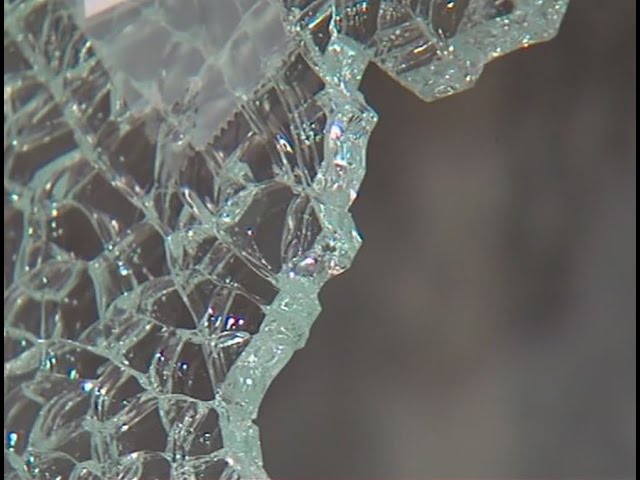The image depicts a highly zoomed-in view of shattered glass. The left side of the picture showcases intricately interconnected shards with numerous small fissures and irregular shapes running through them, giving it an almost crystallized appearance. There is a jagged edge where the glass seems to have been forcefully broken, possibly from an impact like a rock or ball hitting a windshield or window. Interestingly, there appears to be a piece of plastic or scotch tape that spans some of the shards, likely in an attempt to hold the fractured pieces together, with visible ridges on the end. The glass emanates a light green hue, especially noticeable where the light refracts. In the blurry background on the right, shades of gray create an indistinct backdrop, providing no identifiable details beyond the shattered glass.